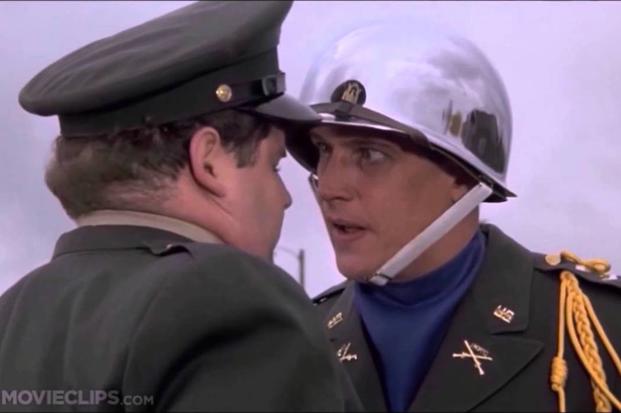The image is a still from the movie "Animal House," featuring two men dressed in military-style green uniforms. The man on the left wears a green parade-style hat, adorned with a gold button securing a green ribbon around the front, and a small black bill. The man on the right sports a chrome-finished metal helmet with a white chin strap, complemented by a yellow ribbon-like adornment on his shoulder, and gold lapel pins showcasing crossed rifles beneath a "U.S." icon. He is also clad in a blue turtleneck under his green military jacket, an unusual choice for a military uniform. The background reveals a cloudy sky, and the image is marked with the watermark "movieclips.com" in white lettering at the bottom left corner.